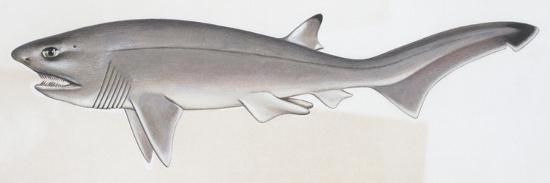This is a small, vintage black-and-white illustration of a shark, likely originating from an old book or scientific journal. The image, measuring approximately 4-5 inches by 3 inches, captures the full body of the shark against a simple cream-colored backdrop, with no indication of water or other fish. The shark is shown in profile with a long oblong body, distinctive striped gills under the head, and inferiorly located fins - two near the front and two towards the back. Its mouth is open, revealing sharp, small teeth, and its eyes appear inaccurately positioned right above the mouth, which is consistent with older, less scientifically accurate illustrations. The tip of the dorsal fin is black, with a small snag, while the rest of the body is predominantly gray. There is a slightly yellowed and reddish hue to the drawing, hinting at its age and possible wear. Despite these imperfections, the illustration emanates a sense of tranquility.